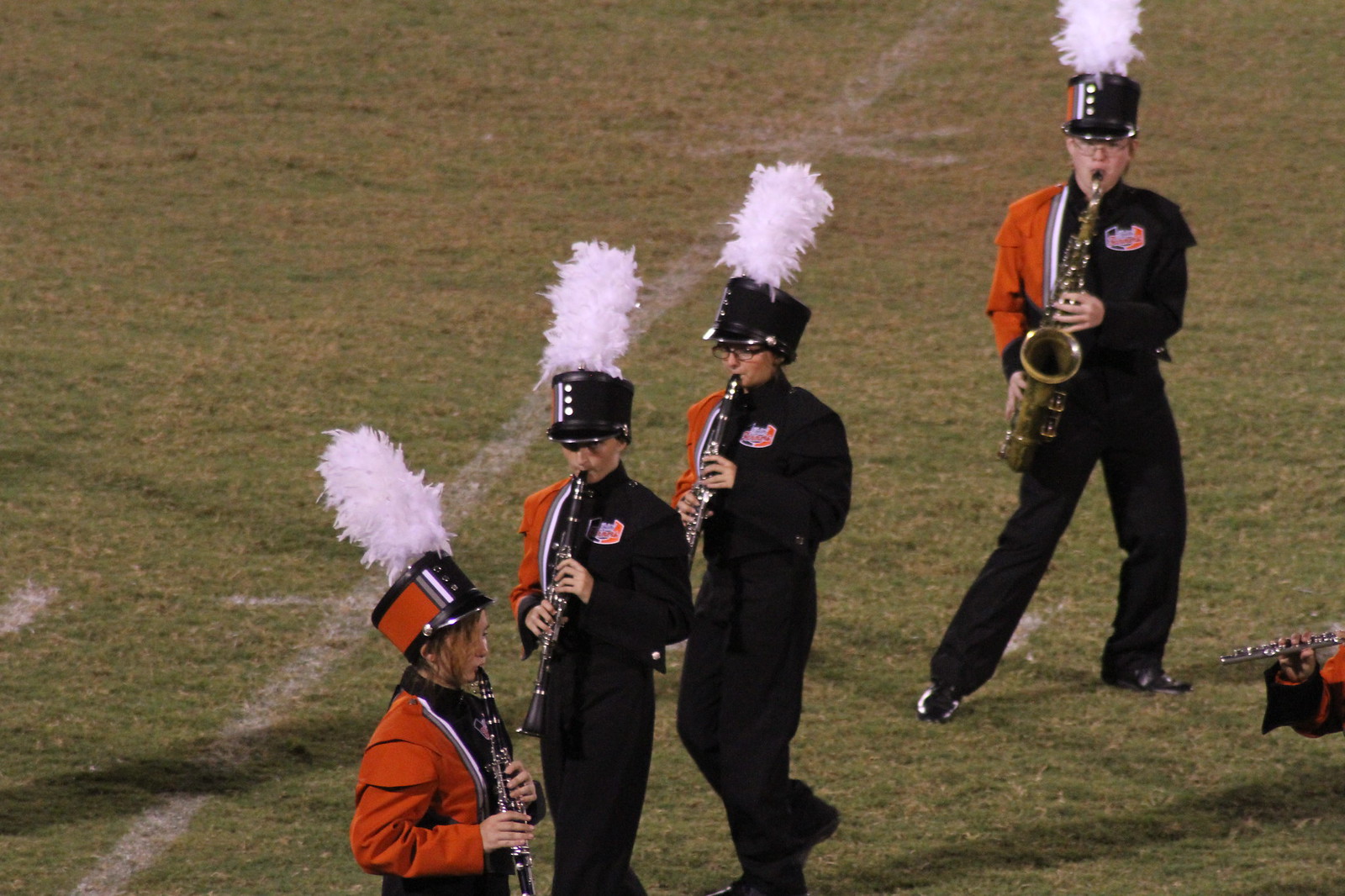This is a detailed color photograph of a marching band, likely from a high school or college, performing on a football field. The image captures four band members in rectangular, horizontal orientation. They are dressed in distinctive black uniforms featuring an orangey-red panel and a white stripe on the right side of their chests and sleeves. Their attire is completed with black shiny shoes and short-brimmed hats, which have an oval vertical siding adorned with three white buttons, and topped with tall white feathers resembling feather dusters.

The scene is set on a lush green football field, visible through the white chalk lines, including a prominent white line extending from the lower left corner upwards. The band members are mid-performance; the player on the far right is playing a saxophone, while the other three to his left are playing clarinets. On the lower right side of the image, there is a partial view of another player, whose hand and flute extend into the frame, hinting at their presence outside the main focus of the shot. There is no text in the image, allowing the viewer to focus solely on the vibrant and dynamic display of the marching band in action.